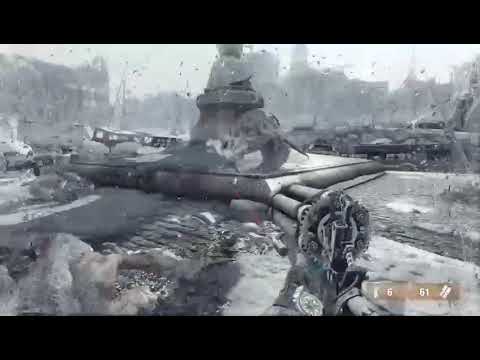This image appears to be a screenshot from a first-person shooter video game, depicting a scene rendered in a monochromatic grey filter that gives it a dark, apocalyptic ambiance. Prominently, the player wields an unusual revolver with six bullets in the chamber and a total of 61 bullets, as indicated in the bottom right corner of the screen. The top and bottom of the screenshot are outlined in black, framing a chaotic urban landscape. The background features a severely damaged cityscape under a grey sky, with a fountain, ruined buildings, and a tank partially visible. In the center of the image is a statue standing on a pedestal surrounded by concrete. To the left of the statue, there appears to be a body of water with some foam. The skyline is brighter on the right side, fading to a dimmer left side, enhancing the overall desolate mood of the scene. Despite the blurriness that obscures some details, the general impression is of a post-apocalyptic or wartime environment, possibly hinting at a fantasy or World War II setting.